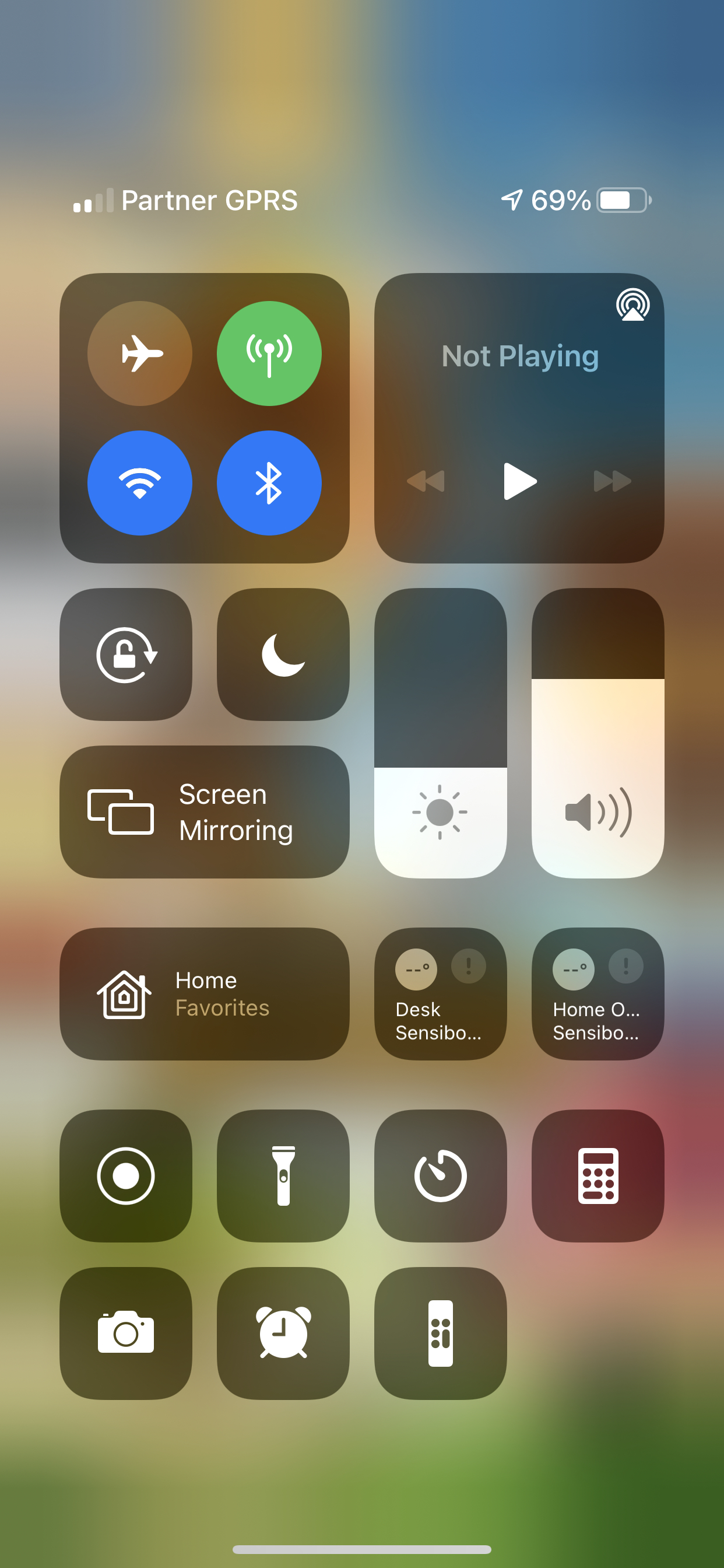Category: Websites

**Caption:**

The image displays a smartphone screen set against a very blurred background. The status bar shows low signal strength and a battery level at 69%. The screen is filled with various apps and options, organized into functional sections.

At the top is a black square housing four clickable icons: Airplane mode, WiFi, Hotspot, and Bluetooth. Right next to it is a video player indicator that currently reads "Not Playing." Below these elements, there's a button for locking the screen. Adjacent to the lock button is another black square featuring a moon icon, which activates night mode.

The screen also features sliders to adjust brightness and volume levels. Additional options include clicking on "Screen Mirroring" and accessing "Home Favorites." Utility icons allow quick access to the flashlight, clock, calculator, camera, and alarm clock. Additionally, there's an icon resembling a remote control, likely intended for operating a TV.